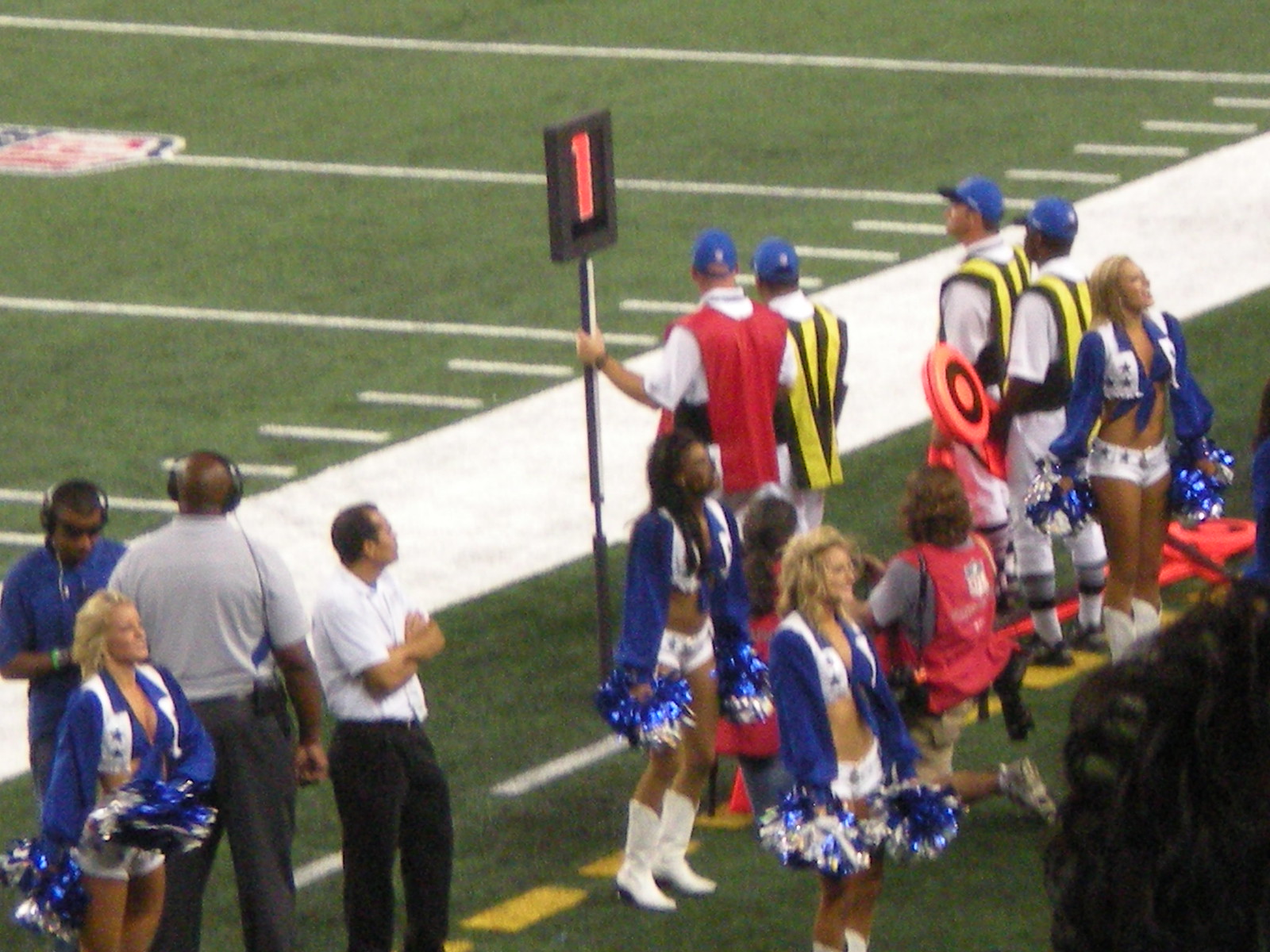In this photograph taken at a football stadium, the sideline is bustling with activity. Five Dallas Cowboys cheerleaders stand prominently, looking towards the crowd. They are dressed in blue, long-sleeve shirts with collars, tied in the middle to reveal their midriffs, complemented by short white vests and white shorts. Nearby, a man in a blue baseball hat wears a red vest and holds a pole with the number 1 indicating a first down.

On the field, referees and officials are noticeable, dressed in black and yellow striped vests, while the green grass is marked with bold white lines. In the top right corner, three gentlemen with blue baseball hats join in the officiating duties. Towards the bottom left, two coaches or staff members equipped with headsets engage in communication, while another individual in a white shirt seems to be observing the scene. A photographer is also kneeling on the ground, capturing the vibrant yet somewhat blurry and noisy essence of what appears to be an older photograph. Despite its age and quality, the image vividly captures the hustle and coordination on the football sidelines.